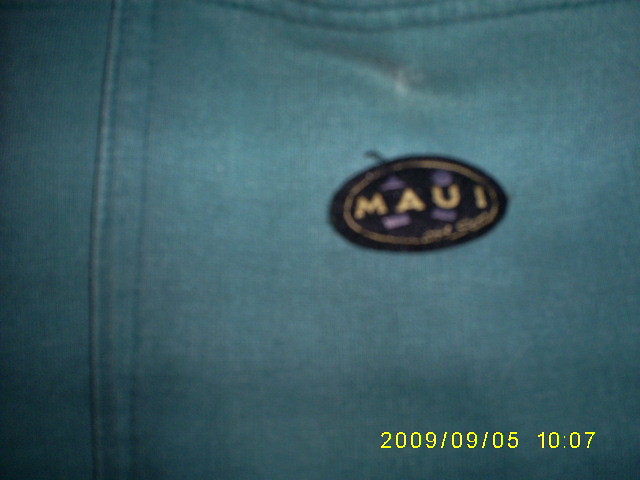This image is a close-up photograph of the back pocket of a pair of blue jeans. The denim is a grayish-blue color and slightly blurry in the image, making the thread texture hard to discern. Superimposed in the bottom right corner is a date stamp: "2009-09-05-10-07." In the left center of the photograph, the seam of the pocket is visible, as well as the top opening of the pocket. Sewn onto this pocket, just below the opening, is an oval black patch. This patch features the word "Maui" in bold yellow text. Additionally, there are purple shapes and more yellow detailing around the word "Maui."